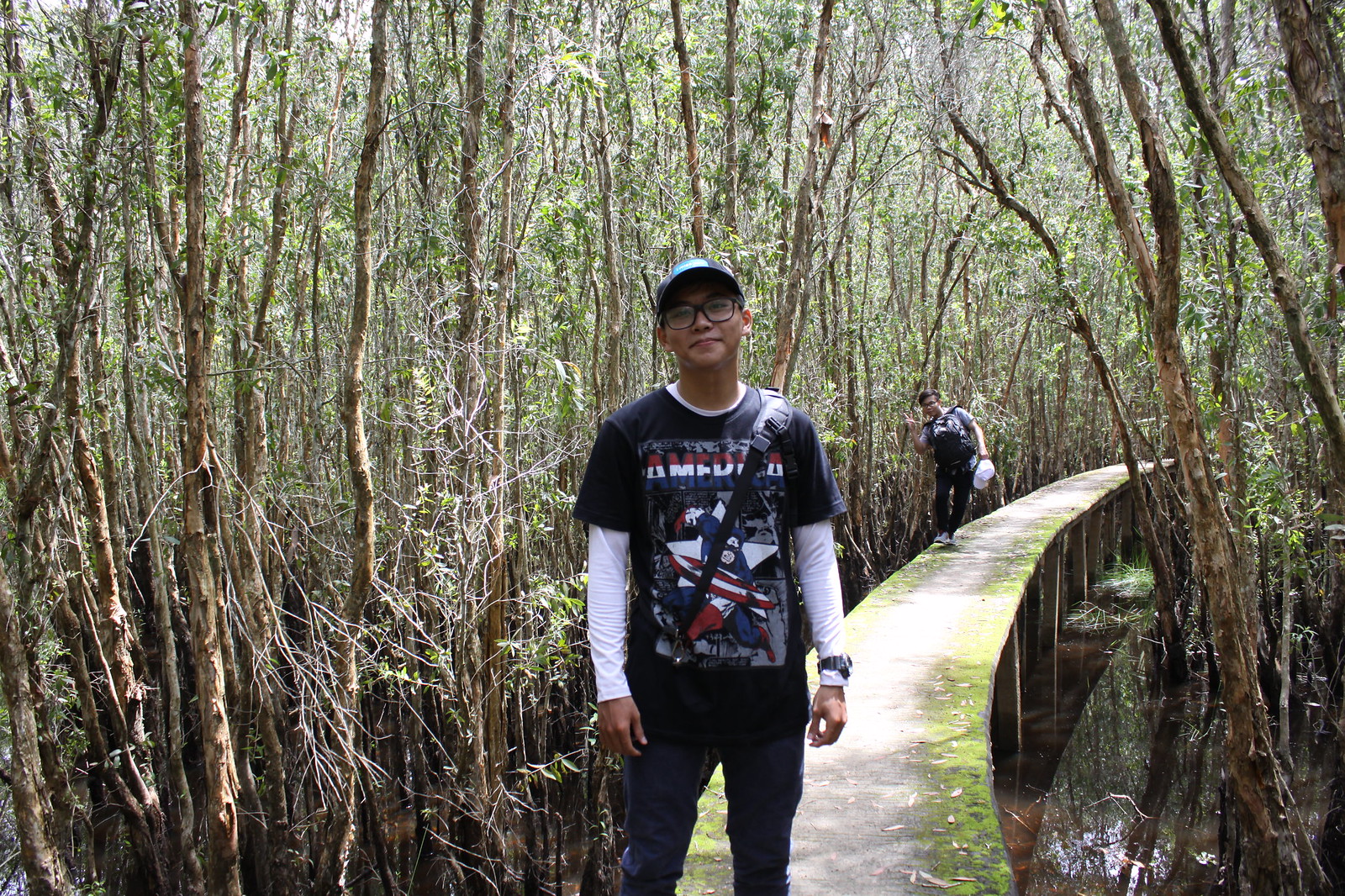This photograph captures two young Asian men walking on a narrow, suspended footbridge with no railings, which appears only wide enough for a single person. The pathway curves from the bottom right of the frame and bends to the right again amidst a densely wooded area with tall, slender tree trunks. Below the bridge, there is a swamp-like body of water.

The man closest to the camera is in his early 20s, wearing a black baseball cap and black-framed glasses. He is dressed in a black t-shirt featuring the word "America" and a graphic of Captain America, layered over a white long-sleeved shirt. He also has on dark pants and carries a satchel over his shoulder. Smiling, he looks forward, appearing happy and relaxed.

A second young man is visible further along the bridge, walking towards the first. This man wears dark pants and holds a white baseball cap in his hand. He has a backpack strapped to his chest and cheekily leans against the bridge as he glances toward the camera, adding a casual and friendly atmosphere to the image. Below the bridge, there is a swampy body of water encircled by tall, slender tree trunks, underlining the natural and rustic setting.